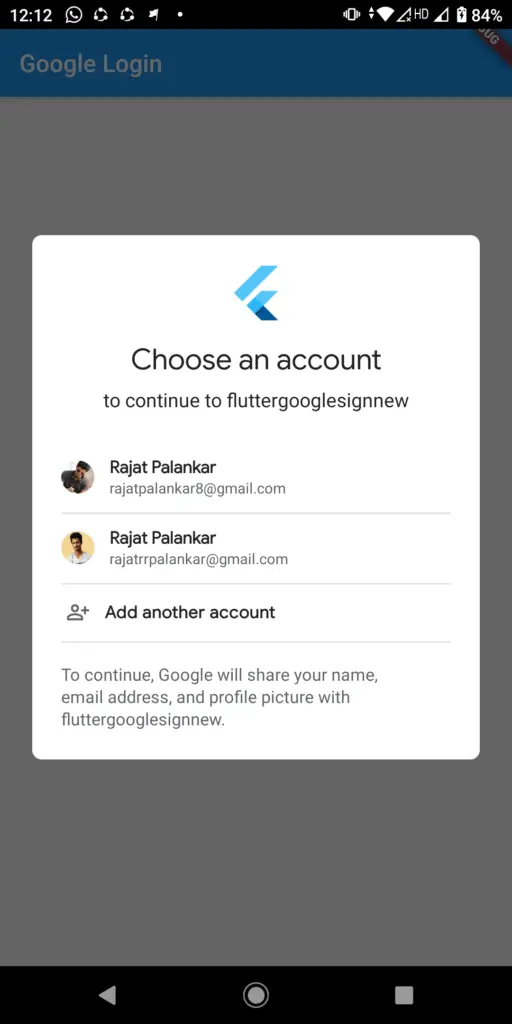A smartphone screen displays a Google login dialogue box, prompting the user to "Choose an account." The dialogue box features a white background with a blue and light blue header. Within the box, two nearly identical email options are listed: "raja.palinkerr@gmail.com" and "raja.palinkerr@gmail.com." Notably, one of the emails has "aid" at the end, while the other does not. Below these options is a link to "Add another account."

A disclaimer text at the bottom informs users that, to continue, Google will share their name, email address, and profile picture with Flutter's new Google sign-in process. At the very top of the screen, the current time, Wi-Fi signal strength, HD icon, and battery life (84%) are displayed. 

Below the main dialogue box, a white area with a blue bar contains a "Google login" button. 

The phone's navigation bar at the very bottom includes three buttons: a back arrow, a home button symbolized by a circle, and an overview button represented by a square. 

The back button navigates to the previous screen while the home button returns to the home screen.